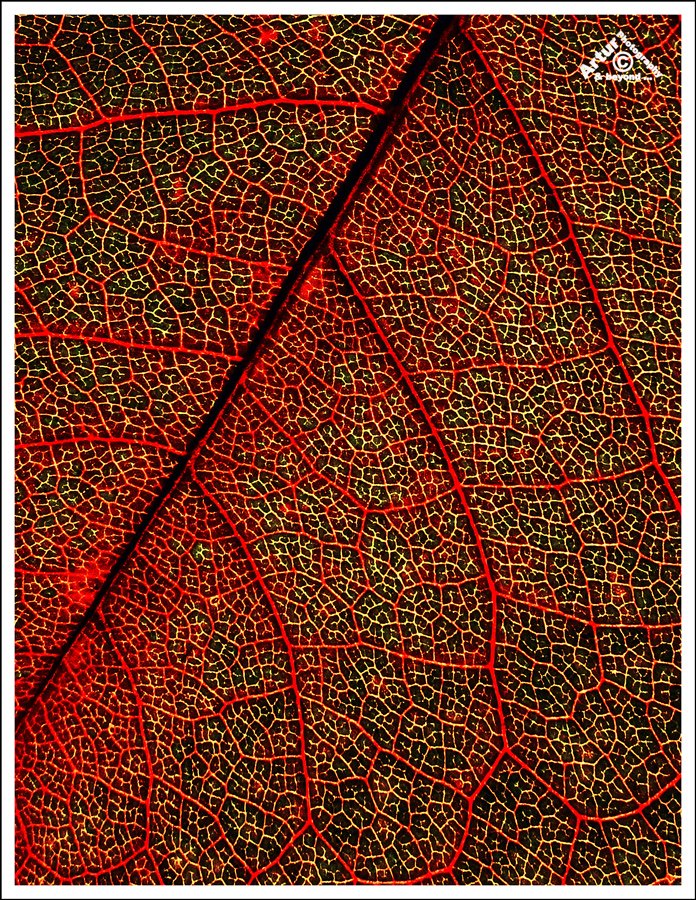This tall, rectangular digital artwork appears to be an extreme close-up, possibly a microscopic view, of a leaf's surface. Enclosed by a black frame with a thin white border, the image showcases a striking and intricate pattern. The color palette includes deep reddish hues, dark purple-black, light yellowish beige, and a dark purple shade. The central vein of the leaf starts near the top, slightly right of center, and descends diagonally to the bottom-left corner. This main vein is a dark red, almost purple-black color, accented by red blobs. Branching from it are thick, curved red veins, creating an elaborate network across the image. Subtle lighter yellowish lines interweave with the more pronounced red veins, suggesting depth and texture. In the top-right corner, there is a white text logo that reads, "ARTUR Photography and Beyond Copyright." The overall aesthetic of the artwork evokes a vivid and detailed portrayal of the leaf, embracing both its natural beauty and its abstract qualities.